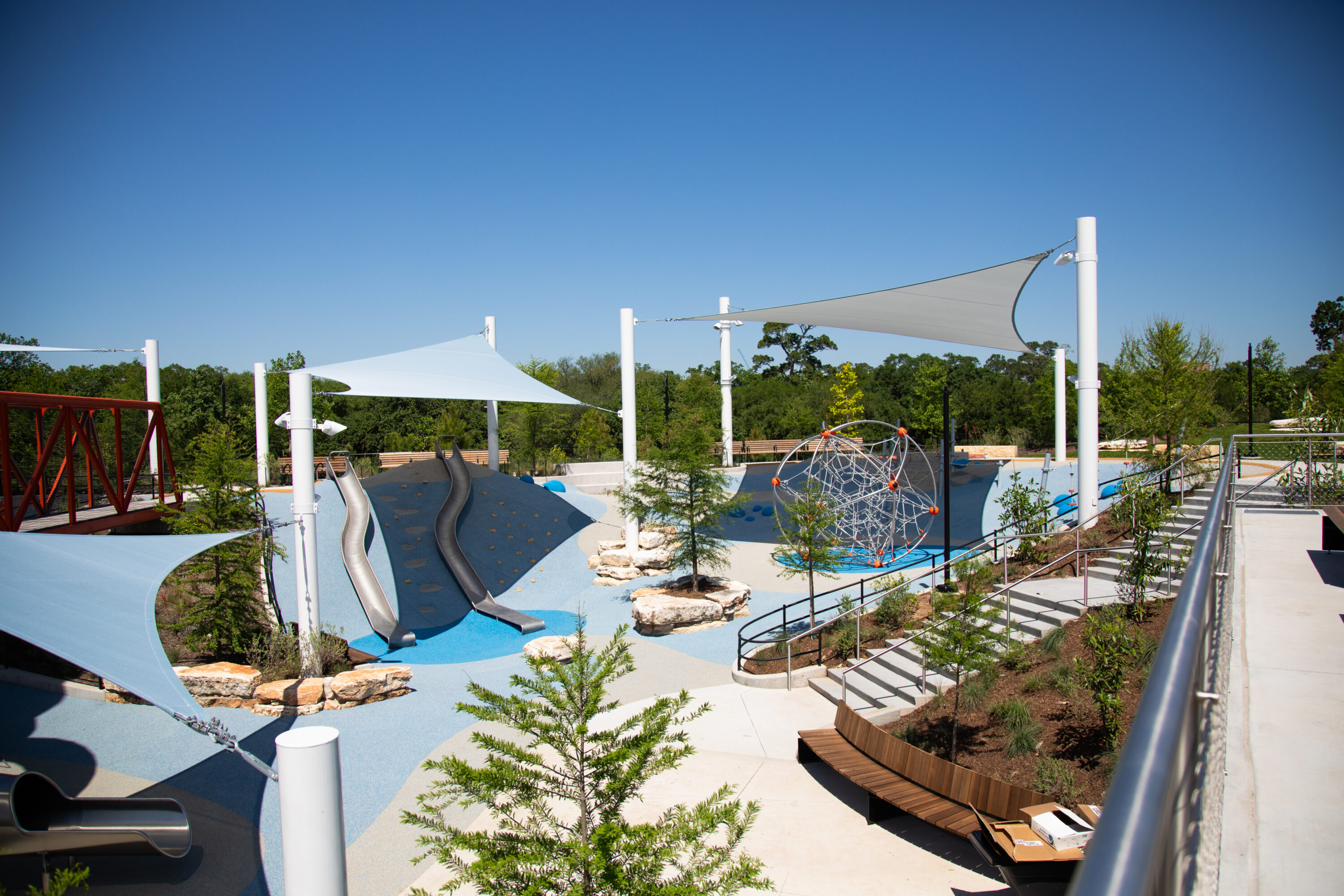This image presents a vibrant playground set in a sunny park. On the right-hand side, there’s a raised porch-like awning with a railing, accessible by a double set of stairs that level off midway. Below this, a wooden bench sits serenely on a curved plane surrounded by trees and bushes. In the bottom left, the exit of a metal tube slide peeks out. Two prominent metal tube slides in the center twist and curve down into a darker blue area. They are shielded from the sun by blue canopies supported by white poles.

Additionally, to the left, another metal slide extends off-frame, while a vivid red bridge adds a splash of color. Nearby, a jungle gym incorporates a spider web-like climbing structure encased in a silver hoop. The playground's surface is mostly blue concrete, interspersed with gardens, young green trees, and a few rock formations.

The park is designed to offer ample shade with various tarps stretched across white poles. The sky above is a clear blue with slight clouds on the horizon, indicating a sunny day. Lastly, a noteworthy feature is a large metal orb with orange balls for children to climb on, contributing to the playground's fun and dynamic environment.